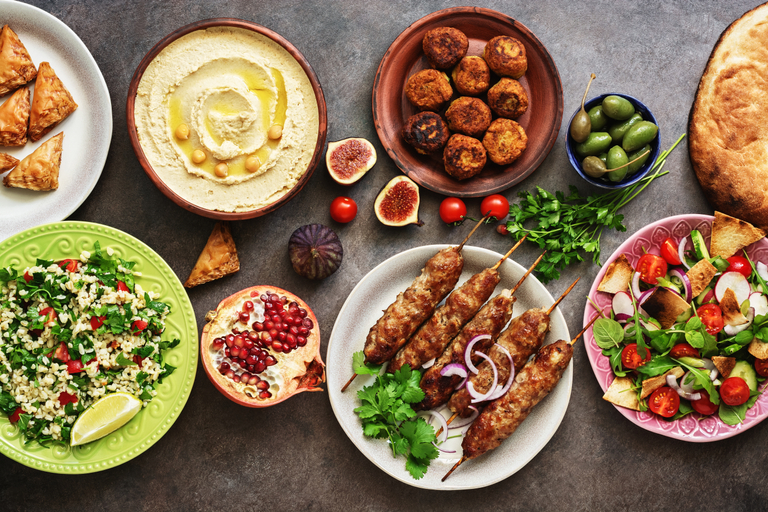This indoor photograph captures a vibrant array of Mediterranean-themed dishes artfully arranged on a textured gray stone countertop with subtle brown accents. The image is rectangular, approximately five inches wide and three to four inches high, with an overhead view presenting two main rows of enticing plates.

In the upper left corner, half of a white plate displays golden-brown triangle pasties. To its right, a round bowl with a dark brown rim holds a spiraled lemon custard garnished with small round balls. Adjacent is another dark brown plate featuring crispy round falafels. Next to this, a small blue plate offers green olives, and a loaf of bread partially enters the frame from the right side.

On the bottom row, a green plate showcases a wedge of lime atop a bed of white grains, red tomatoes, and fresh herbs; likely a spinach tabbouleh salad. Beside this, a halved pomegranate reveals its glistening red seeds. Further to the right, a white circular plate presents chicken kebabs on wooden sticks. The final dish is a pink bowl brimming with a colorful salad of spinach, radishes, cherry tomatoes, and corn tortilla chips.

Interspersed across the table are decorative elements including cherry tomatoes, green herbs like cilantro, another halved pomegranate, and slices of figs showing their reddish-brown interiors. The overall presentation is a feast for the eyes, evocative of the rich and diverse flavors of Mediterranean cuisine.